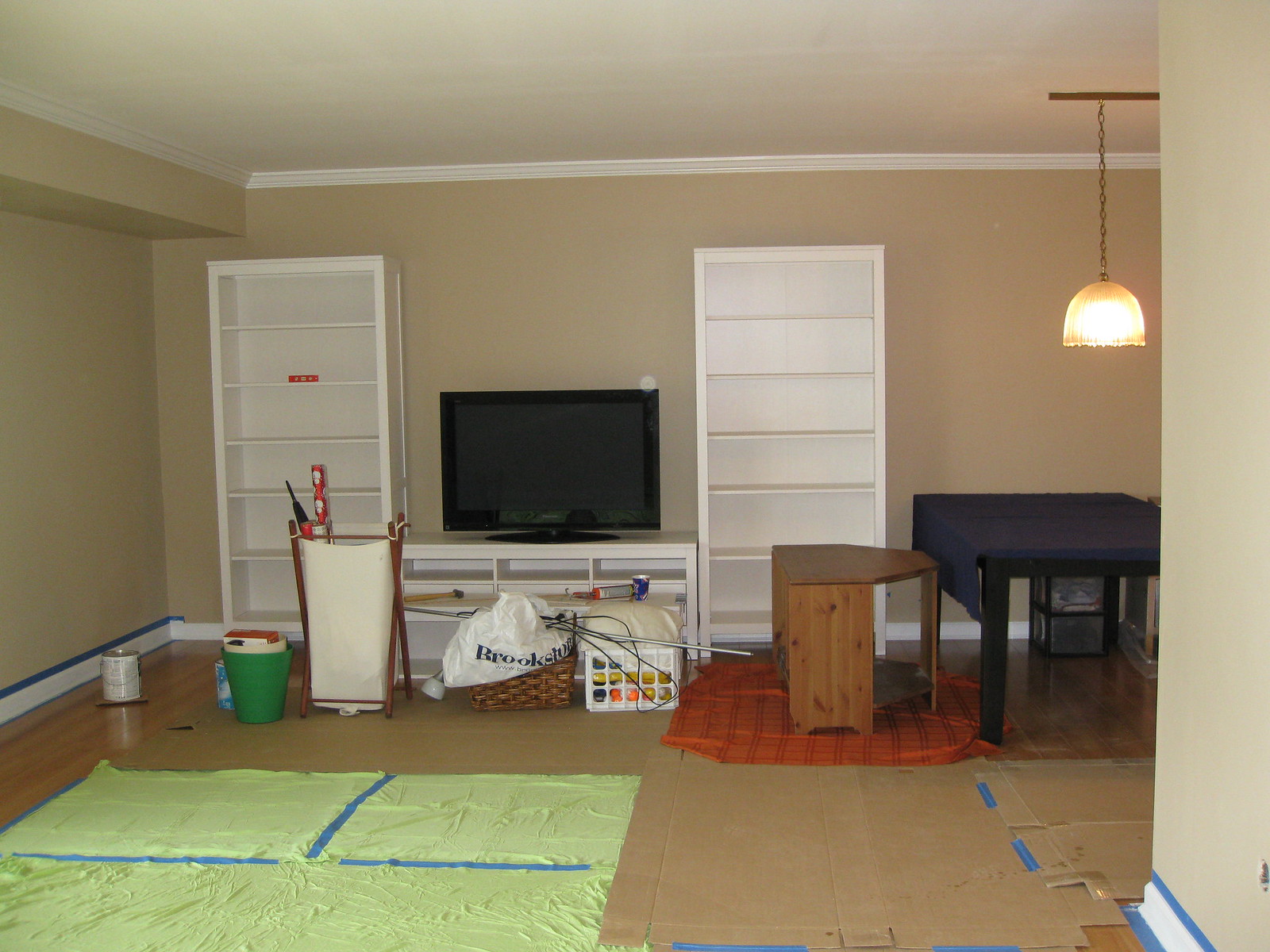This image depicts a room in the process of being prepped for painting. In the right side of the scene, a single lamp hangs from the ceiling. Below it sits a black table draped with a blue tablecloth. Beside this table, an orange blanket featuring red stripes lies on the floor, partially covered by a semi-circular table. In the central part of the room, a white TV stand supports a television, flanked symmetrically by two white bookshelves. The bookshelves and TV stand share a similar design, suggesting they are a coordinated set rather than built-in fixtures. 

Moving further left, the room's floor is fully protected with cardboard and a sheet of green tarp secured by painter's tape. This protective layer extends to the baseboards, which are also masked with painter's tape. Near the center-left are two baskets: one is a laundry basket containing rolls of wrapping paper, and the other is a green basket filled with miscellaneous items. In the back left corner of the room, a solitary bucket of paint stands ready for use. The overall scene captures the careful preparatory steps being taken before the painting process begins.